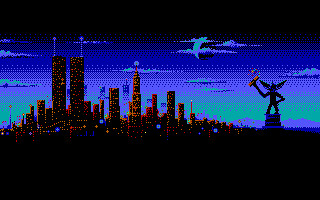A small rectangular image reminiscent of a vintage video game screen, completely pixelated, captures a mesmerizing scene. The top and bottom of the image are flanked by thick black banners, lending a retro aesthetic. Dominating the center-left is a detailed city skyline filled with towering buildings. Each building is illuminated with striking red lights, creating an impression of floors bathed in crimson glow. Adding an element of fantasy, a gremlin statue is positioned towards the left. This gremlin, intricately designed, appears to be holding up a candy cane or a similar type of cane. The background features a moon partially shrouded by clouds, adding an atmospheric touch to this nostalgic digital tableau.